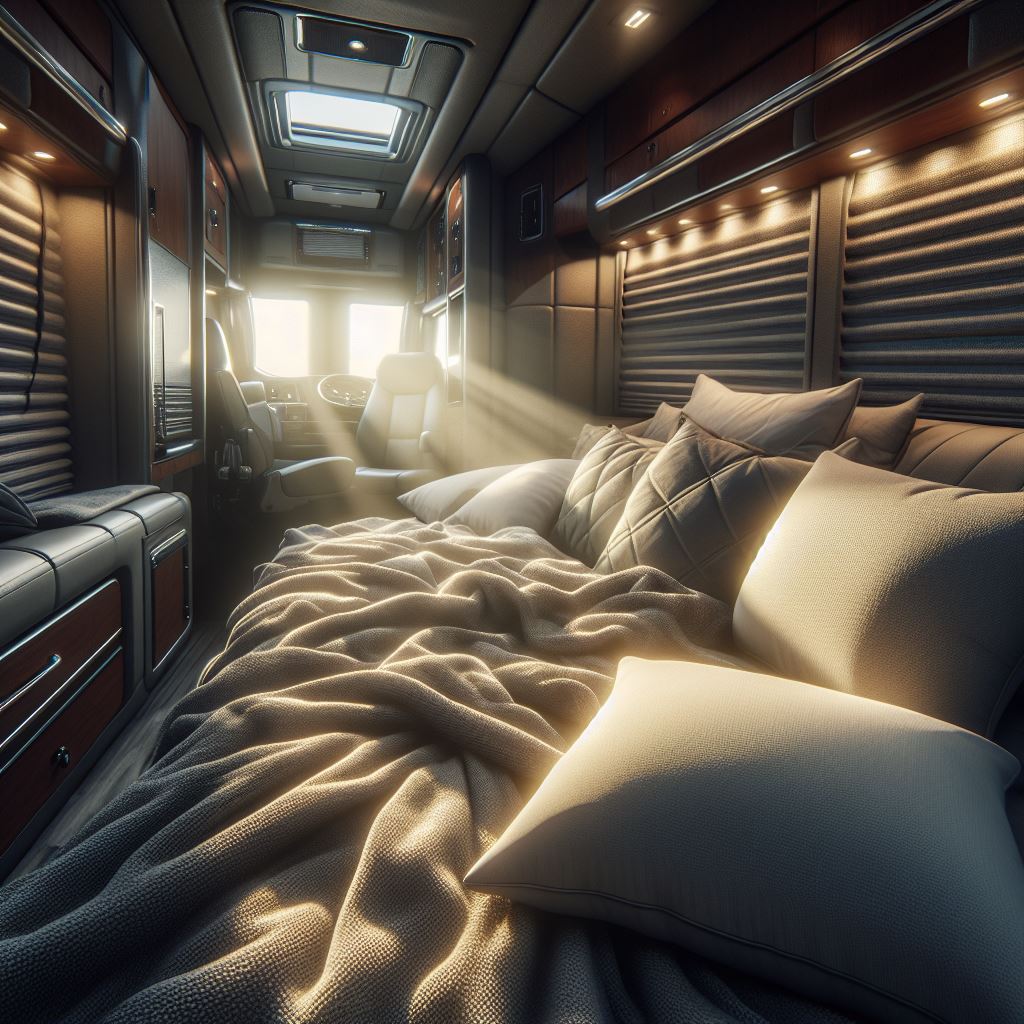This 3D rendering depicts a bright and inviting interior of a luxurious recreational vehicle, bathed in sunlight streaming through the front windshield located at the top left corner of the image. Dominating the foreground is a versatile fold-out bed, originally part of a brown couch, now fully extended and adorned with an assortment of cushions and a cozy, tan Chanel-inspired blanket. The bed features a mix of cushions: two tan, two dark gray pleated, two long white, and three light gray ones leaning against the back of the couch. Flanking this setup, drawn curtains obscure the side windows, adding to the intimate feel of the space. The atmosphere is warmly lit by multiple recessed lights scattered throughout the RV.

In the background, two captain's chairs—one swiveled to face the bed and the other positioned sideways—reside near the driver's area, under a sunroof that lets in additional light. Also visible is a steering wheel near these chairs and a potential leather seat with pull-out drawers or perhaps a mini-fridge to the left side, alongside shaded windows. The beige and taupe color scheme of the interior complements the soft sunlight, creating a serene and refined living space on wheels.